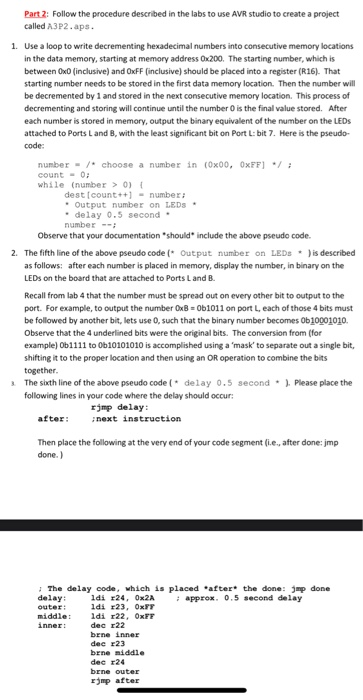This image is a detailed screenshot of a technical website, featuring instructions for creating a project in AVR Studio called "A3P2.APS". The header "Part 2" is prominently displayed in red text and underlined, indicating it is a clickable link. Below, the content is presented in black font.

The instructions guide the user through a procedure from a lab manual. The first step involves using a loop to write decrementing hexadecimal numbers into consecutive memory locations in data memory, starting at address 0x200. It specifies that the starting number, ranging inclusively from 0x00 to 0xff, should be stored in register R16.

The screenshot includes a snippet of pseudocode for this process:

```
number = /* Choose a number in (0x00, 0xff) */;
```

Additionally, the second instruction directs the user to output a number on LEDs, referencing the pseudocode:

```
/* Output number on LEDs */;
```

Further down, the image displays coding output and a section labeled as "delay code," which is to be implemented after the "done, JMP done" instruction. The delay sequence is broken down into outer, middle, and inner loop components, emphasizing precision and technical detail.

Overall, the image provides a comprehensive and intricate example of assembly language programming and embedded systems design.